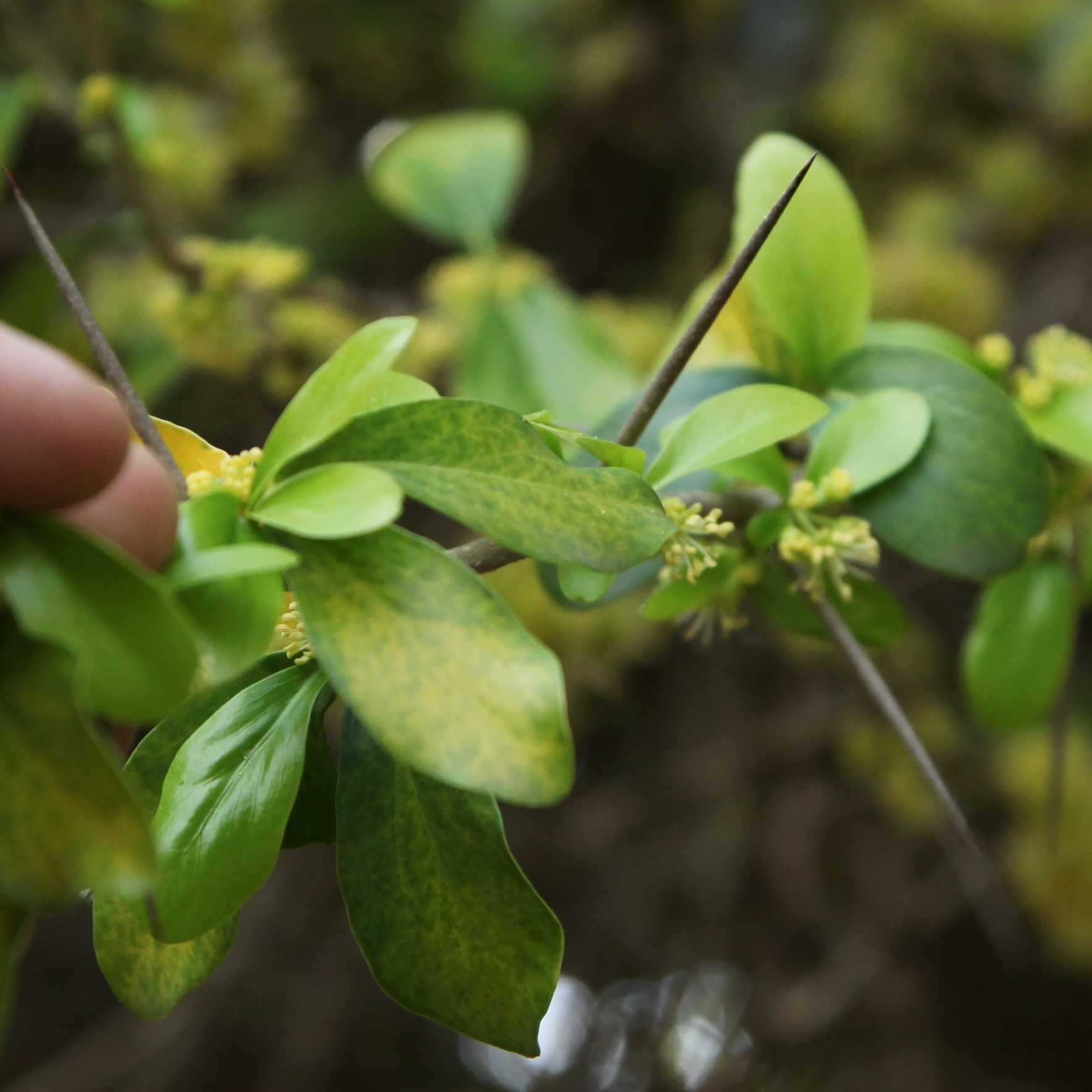In the foreground of this image, two fingertips are gently touching a vibrant, green plant. The plant is adorned with numerous green and yellow petals radiating from its center, which is a prominent yellow hue. Surrounding the focal plant, multiple similar plants can be seen in the slightly blurry background, suggesting a lush and verdant environment. The ground beneath the plants is a dark gray shade, likely due to the presence of soil or dirt. At the very bottom of the image, blurry white circular shapes are visible, though their exact nature is unclear. The plant in the center exhibits gray, needle-like spikes or stems extending from both its left and right sides, adding an intriguing and slightly mysterious element to its appearance.